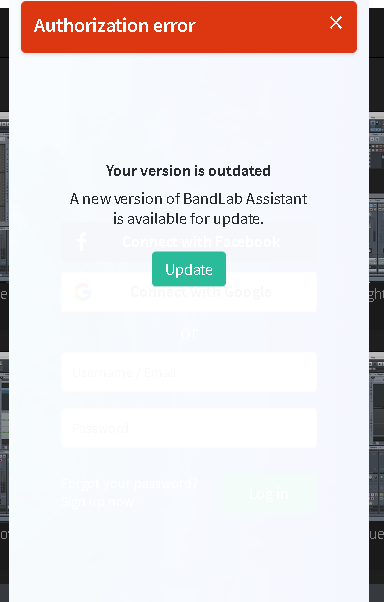The image is a screenshot taken from a smartphone, showcasing a significant white pop-up box dominating the center of the screen against a black background. This pop-up is almost as large as the phone's display. At the very top of the pop-up, there is a red rectangular box with the text "Authorization Error" written in white letters, accompanied by an 'X' on the right side for closing the notification.

Below this, the main section of the pop-up has a white background with a message stating, "Your version is outdated. A new version of BandLab Assistant is available for update." Towards the bottom of the pop-up, there is a smaller green rectangular box containing the word "Update" in white letters.

Through the semi-transparent pop-up, parts of the underlying screen are faintly visible. This includes a Facebook logo with the text "Connect with Facebook" and a Google logo with the text "Connect with Google." Additionally, two empty white text boxes can be seen, likely intended for entering a username and password. There is also another green button to the right, partially obscured by the pop-up.

In the black background behind the pop-up, there are subtle gray marks and patterns, though their exact nature is unclear due to the focus on the central white pop-up box.